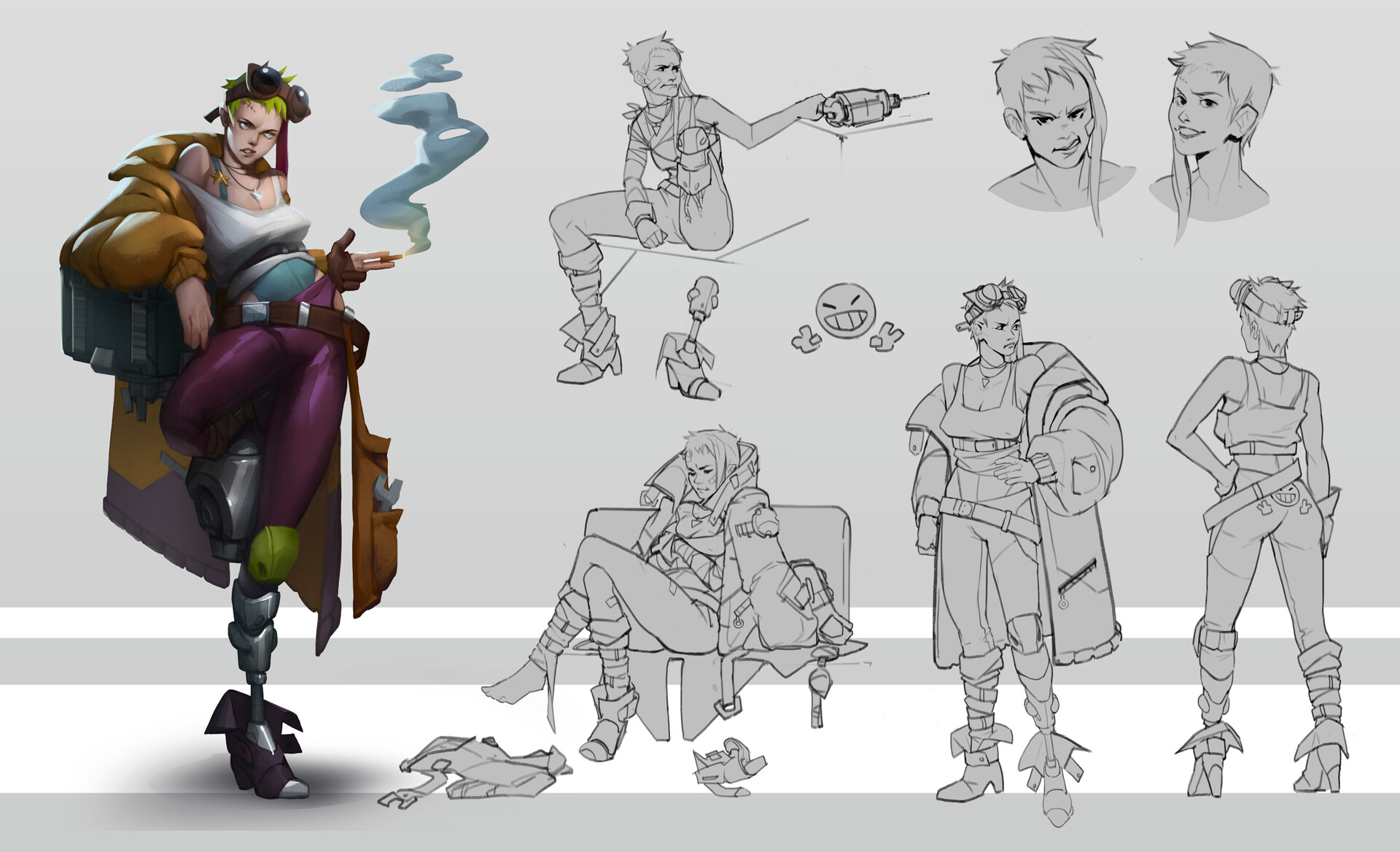The image is a detailed piece of concept art, predominantly in shades of gray and black, depicting various sketches of a female character, with one full-color drawing of her on the far left. This central figure is adorned in striking attire: she sports green hair beneath a brown pilot's hat with hanging straps, a white sleeveless top, a bulky brown coat with a blue accessory draped from it, purple pants, a brown belt, and metallic spiraled legs that end in purple heels. A cigarette with blue smoke is held in one hand. The monochrome sketches surrounding her display different views and poses. One full-body sketch is in the upper right, two headshots with differing expressions are nearby, another shows her seated on a bench and removing her legs with a drill next to her, and yet another presents a rear view sans coat, revealing her detailed mechanical legs and top. The background is a mix of light blue with white at the bottom, lending an air of cohesiveness to the character's varied portrayals and phases.